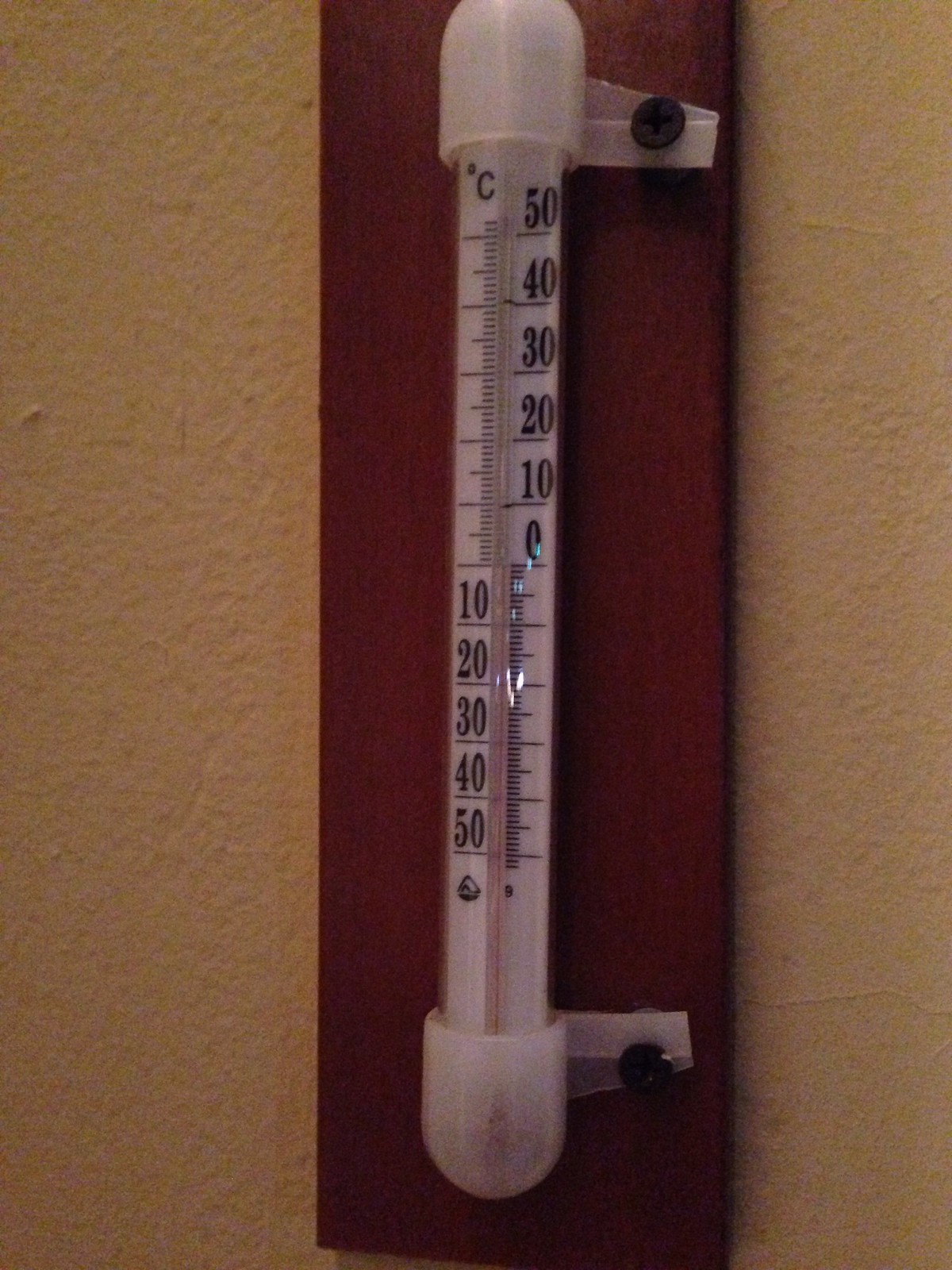The image captures a thermometer mounted on a wooden slab affixed to a wall. The thermometer, which is predominantly white with black text and markings, measures temperature in Celsius. Its scale is split in the middle, displaying positive temperatures from 0 to 50 degrees Celsius on the right-hand side and negative temperatures from 0 to -50 degrees Celsius on the left-hand side, though no negative markings are visible. 

At the base of the thermometer, below the negative scale, there is a triangular emblem resembling a tent, hovering above a round, cylindrical foundation that likely serves as the manufacturer's logo. The temperature reading on the thermometer is difficult to discern, with a thin red line indicating a position around 0 degrees Celsius.

The thermometer is secured to the wooden slab with two black screws, encased in white, oval-shaped holders positioned at the top and bottom. The overall structure is mounted perpendicular to the frame. The background wall behind the wooden slab is composed of tan to beige drywall, showing some wrinkles and minimal imperfections, particularly noticeable in the bottom right-hand corner of the image.